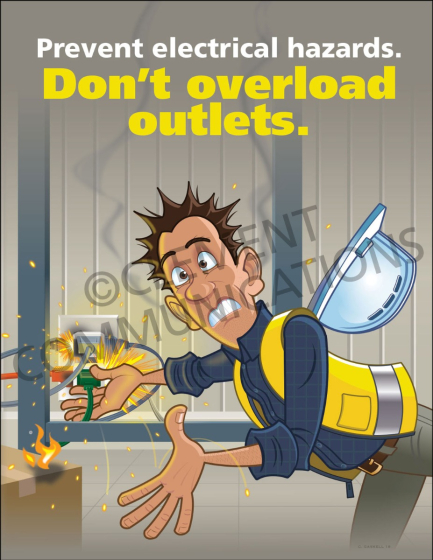This vibrant comic-style safety poster features a panicked construction worker with his hair spiked up, appearing to be electrocuted. He is wearing a yellow safety vest over a blue long-sleeved shirt with rolled-up sleeves, khaki work pants, and a brown belt. His hard hat is slipping off his head as he plugs into a heavily overloaded electrical outlet, which is emitting dangerous flames and sparks. The outlet, already crowded with white, red, and blue plugs, highlights the hazardous mistake. The scene is set against light brown walls, suggesting an indoor environment. Prominent text at the top warns "Prevent Electrical Hazards" in white, while bold yellow letters below command "Don't Overload Outlets." Additionally, there is a watermark in the middle of the image, identifying it as copyrighted by Cement Communications.